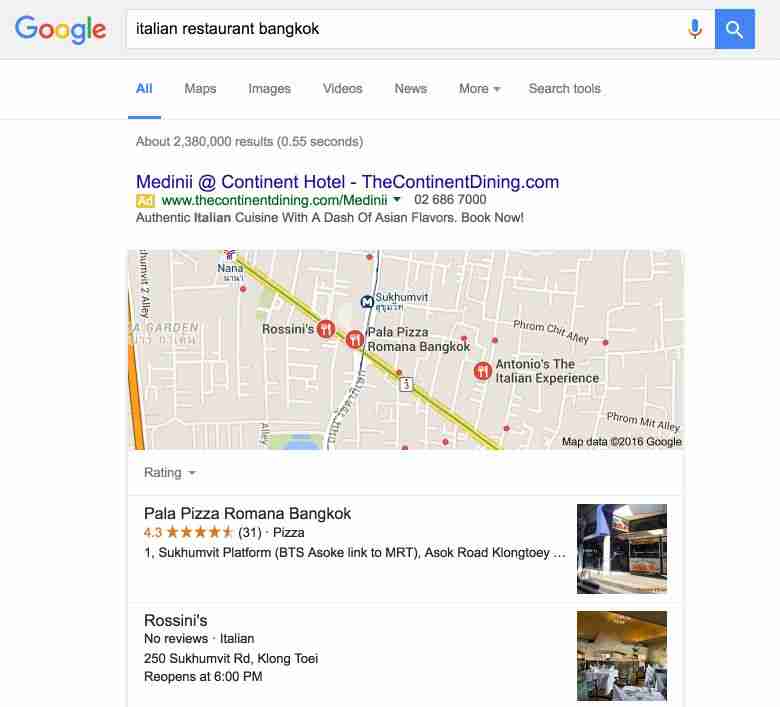The image depicts the results of a Google search for "Italian restaurant Bangkok." In the top-left corner, the iconic Google logo is visible. Below it sits a white search bar with the query "Italian restaurant Bangkok" entered. The search returned approximately 2,380,000 results in just 0.55 seconds.

At the top of the search results appears an advertisement from "Medini at Continental Hotel" hosted on the website thecontinentdining.com. It features a small "Ad" label, a phone number for reservations, and a brief description: "Authentic Italian cuisine with a dash of Asian flavors. Book now!" Alongside the ad, a map highlights the restaurant's location.

Further down, the results include a list of other Italian restaurants in Bangkok. "Pala Pizza Romana Bangkok" boasts a 4.3-star rating. In contrast, "Rossini's" is featured without any reviews. Accompanying these entries are two small thumbnail images showing the interiors of these two Italian eateries.